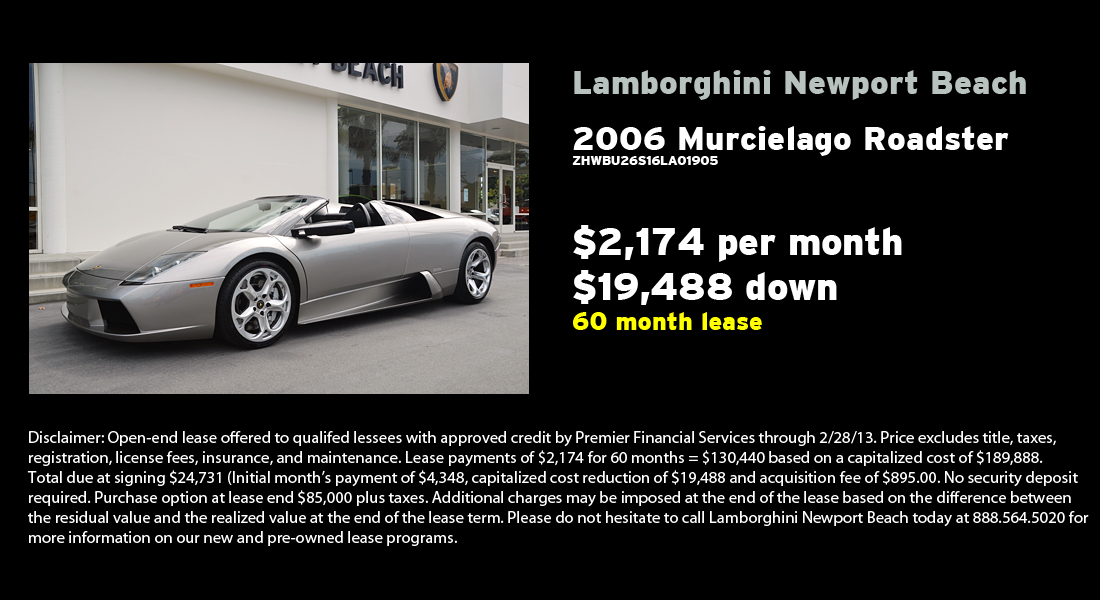The advertisement, set against a sleek black background, showcases a silver 2006 Lamborghini Murciélago Roadster without a roof, parked next to a shop with a white wall, glass window, and a glass entrance door, highlighting a short flight of stairs leading to the door. "Lamborghini Newport Beach" is prominently displayed in white text on the right, followed by details of the lease: $2,174 per month with a down payment of $19,488 for a 60-month term, the latter highlighted in yellow. Below these details, a paragraph of fine print provides further terms and conditions.